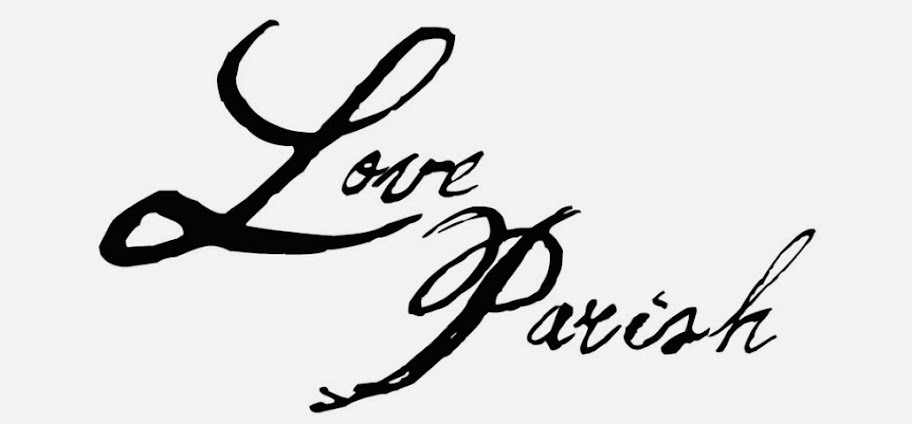The image is a long, rectangular piece featuring an off-white, almost light gray background with no border. The focal point is text in a solid black, highly decorative script that mimics hand-painted brushstrokes, although it is more likely digitally created. At the top, the word "Love" is prominently displayed with an especially large and dramatic "L" that curves dynamically to the right. Below and slightly to the right, "Parrish" follows, with a similarly extravagant "P" that matches the style of the "L." Together, the text forms "Love Parrish," possibly suggesting a name for a store or design company. The entire design is free from illustrations, photographs, or brand markings, evoking the look of an elegant, boutique sign.